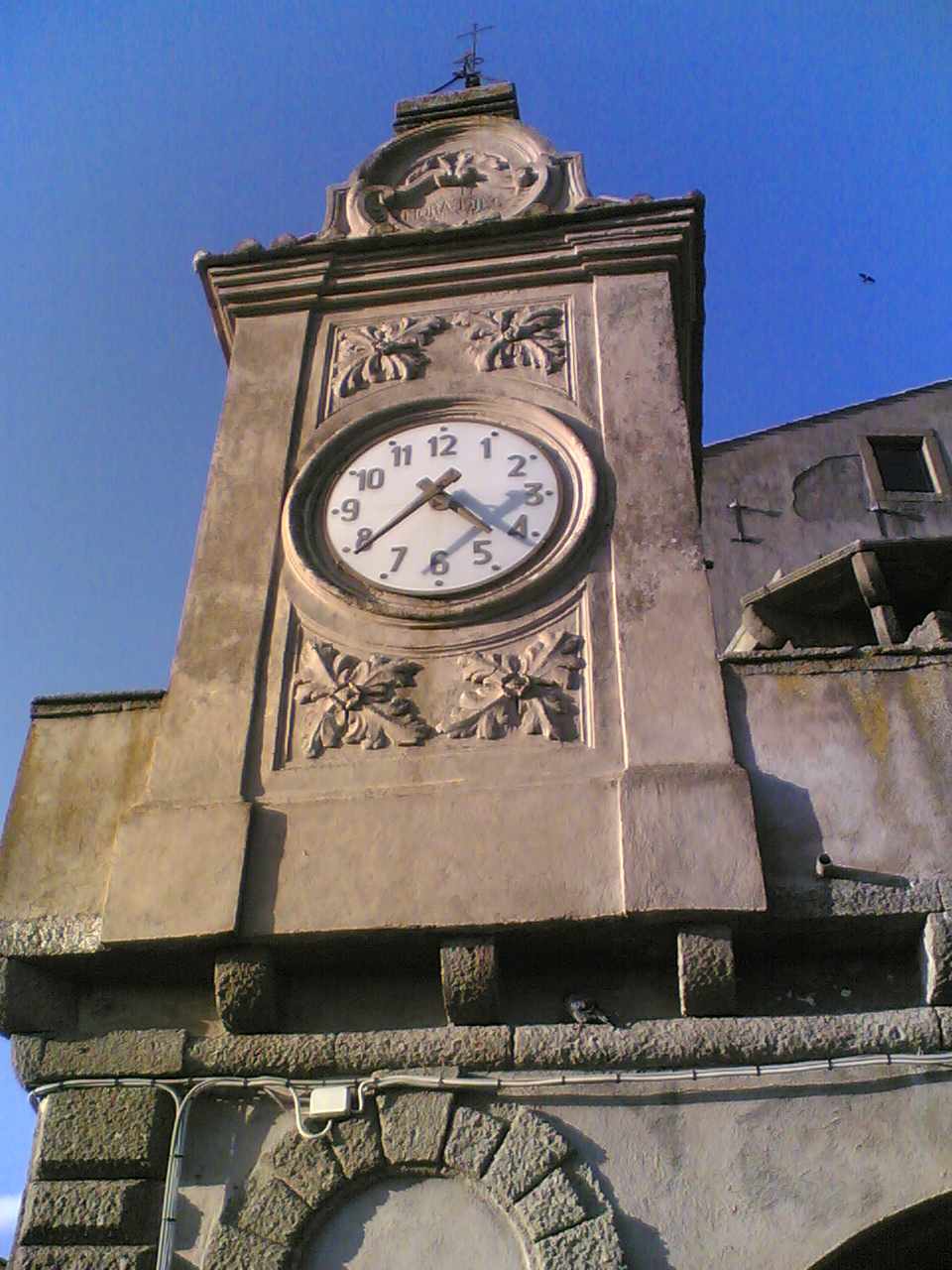This captivating image showcases a magnificent clock adorning the exterior of an imposing, ornately designed tower. The structure, composed of cement and adorned with intricate brickwork and arches, exudes a majestic architectural charm. The large rectangular section housing the clock is embellished with two ornate leaf designs above and two below. Crowned at the top of the rectangle is a distinctive circular motif that adds to the tower's grandeur. The clock itself features a white face with brown numerals, the hands also constructed in brown, indicating the time as approximately 4:39. To the right of this exquisite building, a square notch resembling a window is visible, accompanied by areas exhibiting signs of rust, contributing a touch of rustic character to the scene.